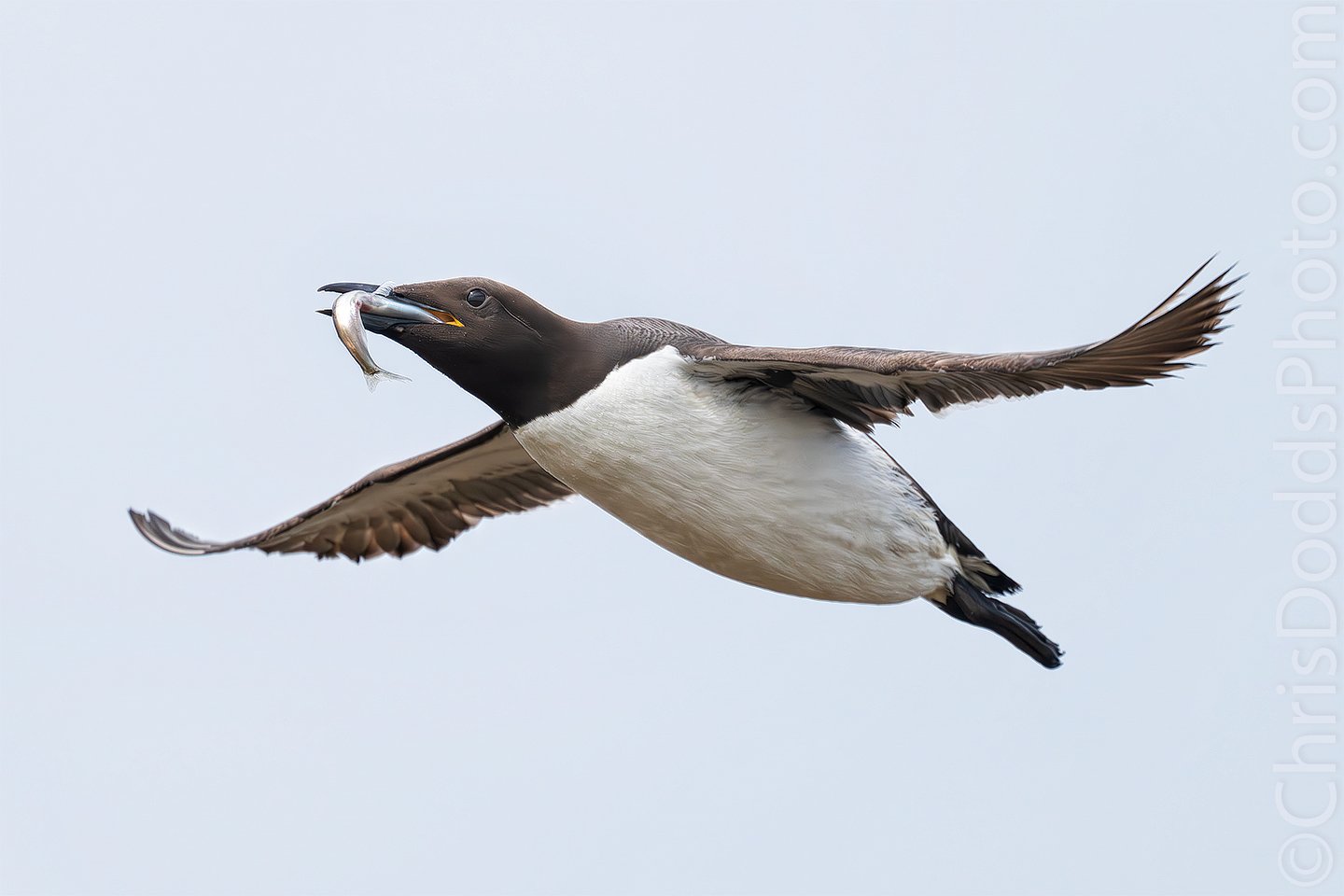This color photograph captures a large seabird in mid-flight against a light gray sky. The bird is characterized by its striking black head, back, wings, and tail, contrasted by its white belly and chest. Its outstretched wings display a hint of white outline. The bird's black feet are visible, adding to the distinct color pattern. A closer inspection reveals a beady black eye and a partially open beak, tightly gripping a silver fish, with the fish's tail curving downwards and to the right. The bird is angled in such a way that its body faces left in the image. There is a subtle, transparent watermark in the bottom right corner that reads "chrisdoddsphoto.com."